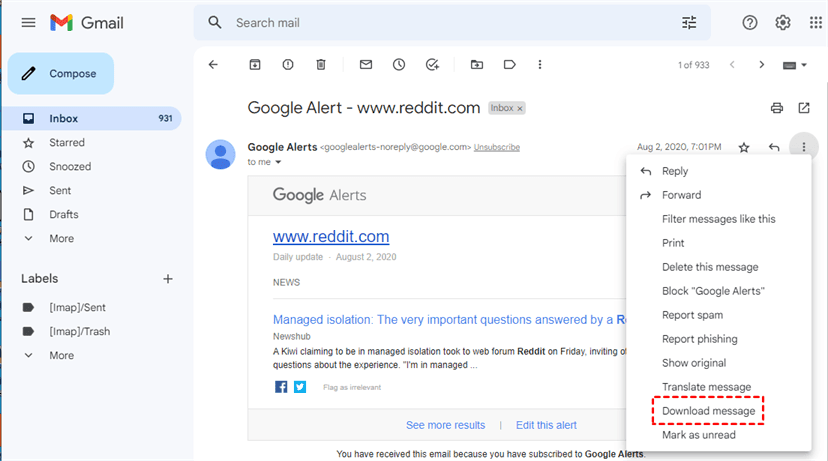This detailed screenshot from the Gmail web interface captures a user's inbox page. Dominating the left side is a vibrant, multi-colored sidebar that features the familiar Gmail icon, a prominent blue "Compose" button, and several mailbox categories including "Inbox" — which is currently highlighted and showing a total of 931 messages.

The user interface also displays other categories such as "Starred," "Snoozed," "Sent," "Drafts," and a "More" dropdown that reveals additional labels including "IMAP Sent" and "Trash." At the top, there's a search box with various icons, including a gear icon for settings located towards the right.

Below the search bar is a line of smaller icons alongside a Google Alerts email in the inbox. This email is marked with a small round Google icon next to a blue head-and-shoulders symbol, indicating the sender is "Google Alerts" from the email address noreply@google.com. The subject line reads, "reddit.com daily update August 2, 2020," containing news updates. One of the highlighted updates within the email mentions “Managed isolation: The very important questions answered by AR,” with a partial preview of content describing how a person in managed isolation shared their experience on a web forum.

To the right, a pop-up menu obscures part of the screen, offering options such as "Reply," "Forward," "Filter messages like this," "Print," "Delete this message," "Block Google Alerts," "Report spam," "Report phishing," "Show original," and "Download message." This menu is outlined in a broken red rectangle, with red markers at the bottom indicating that it's a screenshot intended for instructional use, possibly showing someone how to download the message.

The overall image provides a clear, instructive view of navigating and managing the Gmail web interface.